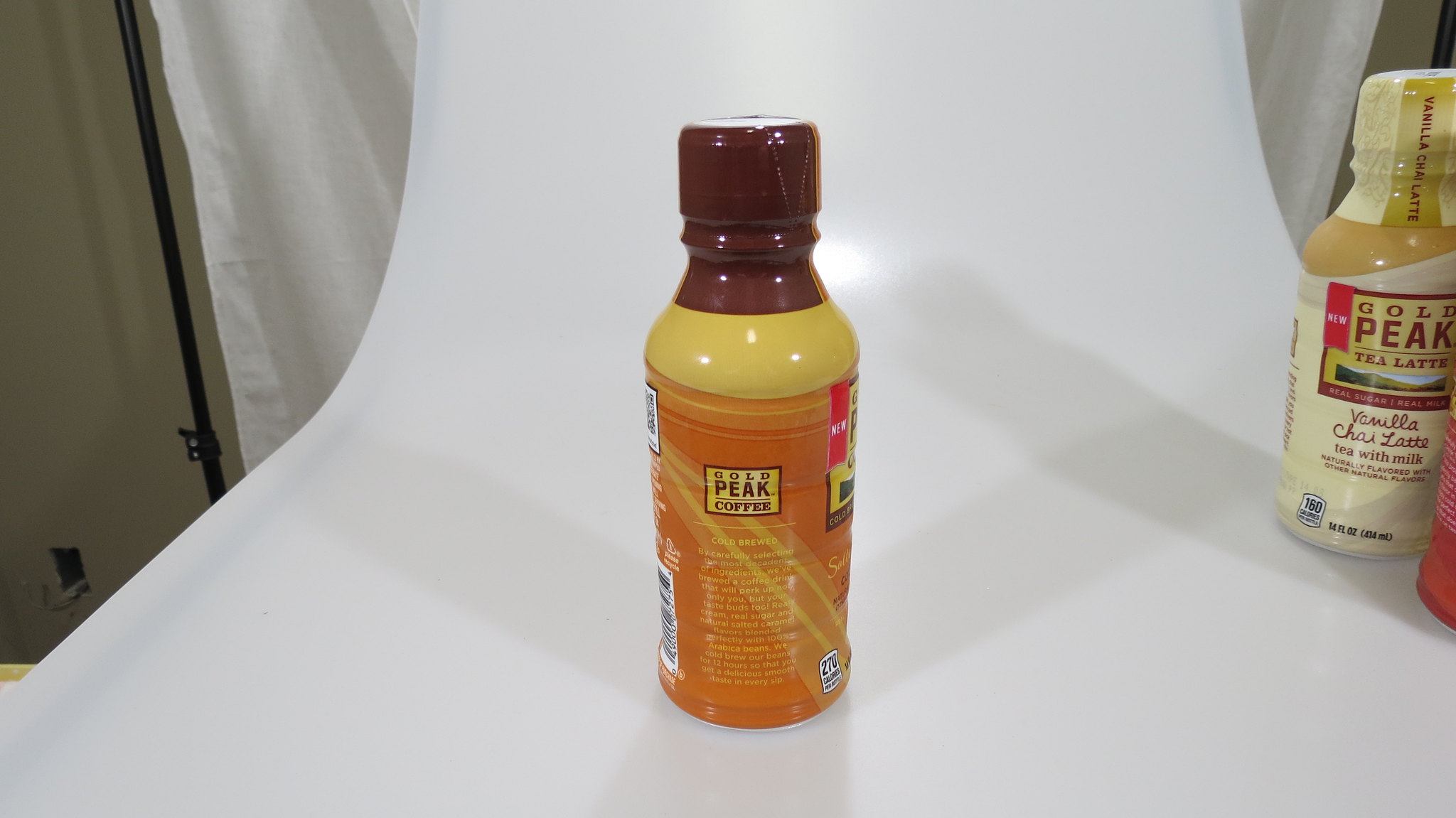This image captures a professional photo shoot setup featuring Gold Peak beverages. The backdrop consists of elegant white drapes, creating a clean and polished aesthetic. Centered in the composition is a Gold Peak Coffee bottle, distinctly plastic with a sealed lid. To its right, a Gold Peak Vanilla Chai Latte is positioned, adding variety to the collection. Another bottle is partially visible, indicating the presence of more Gold Peak products in the scene. The meticulous arrangement and high-quality presentation suggest a carefully orchestrated effort to showcase these beverages in the best possible light.